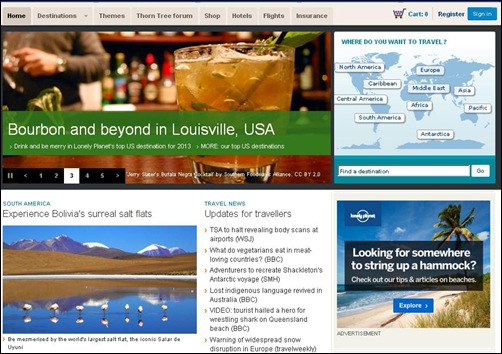This image is a detailed screenshot of a well-designed travel-focused web page. At the top, there is a beige-colored banner featuring various navigation options, among which "Home" is highlighted. The other options listed are Destinations, Themes, Thorn, Free, Forum, Shop, Hotels, Flights, Insurance, Cart, Register, and Sign In.

The main content of the page includes a photograph of a glass of bourbon placed on a polished wooden surface. Behind the bourbon, there is a partial view of a person and shelves stocked with various liquor bottles. A green banner labeled "Bourbon and Beyond in Louisville, USA" is prominently displayed, although the white text beneath is too small to be legible.

To the right of the green banner, a section titled "Where do you want to travel?" lists various global destinations: North America, Caribbean, Central America, South America, Europe, Middle East, Asia, Africa, Pacific, and Antarctica. There’s a prompt below to "Find a destination."

Further down, there is a picturesque photograph of a lake with numerous white birds standing in the water. The lake reflects nearby mountains and a brown, grassy area in the background. This section is captioned with "South America, experience Bolivia's surreal salt flats" and includes a description inviting visitors to be mesmerized by the world's largest salt flat, the iconic Salar de Uyuni.

Below are various travel news updates, including significant headlines:
- "TSA to halt revealing body scans at airports," Wall Street Journal.
- "What do vegetarians eat in meat-loving countries," BBC.
- "Adventurers to recreate Shackleton's Antarctic voyage," SMH.
- "Lost indigenous language revived in Australia," BBC.
- "Tourist hailed a hero for wrestling shark on Queensland beach," BBC.
- "Warning of widespread snow disruption in Europe," Travel Weekly.

In the bottom-right corner, there's a photograph of a beach adorned with palm trees. The caption reads, "Lonely Planet, looking for somewhere to string up a hammock? Check out our tips and articles on beaches, explore." Directly beneath this photograph, the word "Advertisement" is marked clearly.